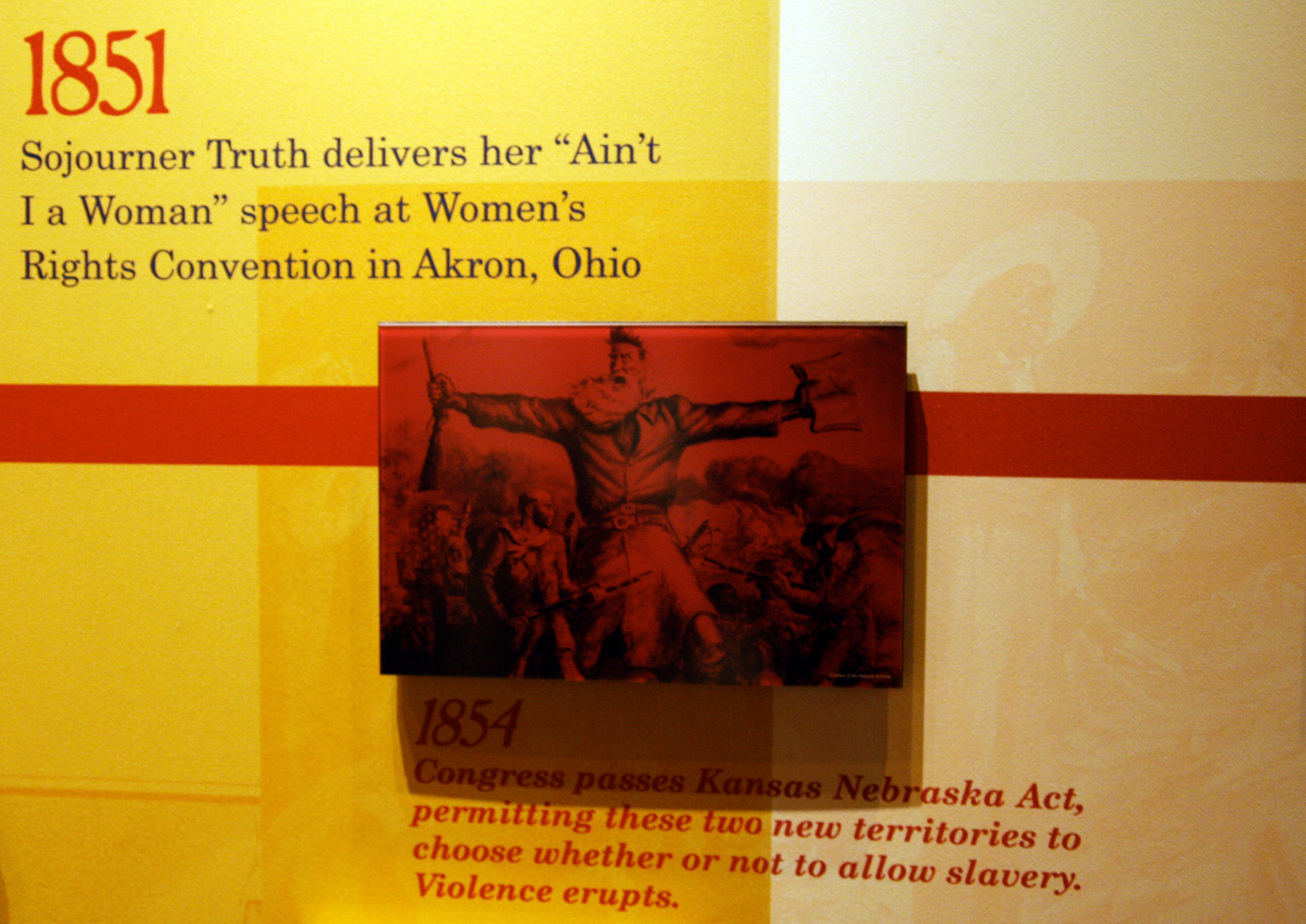The image features a detailed, museum-style artwork displayed against a dual-colored background: yellow on one side and tan on the other, overlaid with faint decorative patterns. In the top left corner, the red text reads "1851," followed by black text stating, "Sojourner Truth delivers her 'Ain’t I a Woman' speech at Women's Rights Convention in Akron, Ohio." Dominating the center of the piece is a striking depiction of a tumultuous scene: a man stands with arms outstretched, holding a book in one hand amidst chaos, characterized by stark red and black tones. Below this illustration, additional text notes, "1854, Congress passes Kansas-Nebraska Act, permitting these two new territories to choose whether or not to allow slavery. Violence erupts." This comprehensive visual narrative highlights the significant events of 1851 and 1854, juxtaposing Sojourner Truth's pivotal speech with the contentious enactment of the Kansas-Nebraska Act.